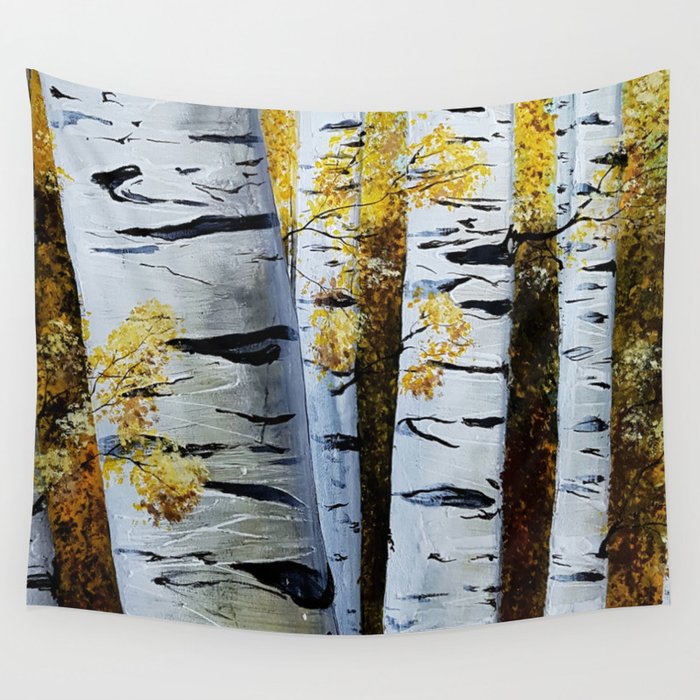The image showcases a square tapestry hanging on a white wall, portraying a painted depiction of white birch trees adorned with yellow and brown leaves. The focal point features a thick, slanted birch tree on the left, marked with characteristic gray and black horizontal stripes, signifying its birch nature. To the right, three slimmer birch trees stand further in the background, each similarly adorned with black stripes and surrounded by small branches of yellow leaves. The tapestry, designed in an artistic painted style, is suspended from its top corners, creating a slight droop in the center, highlighting the detailed and textured portrayal of the forest scene.